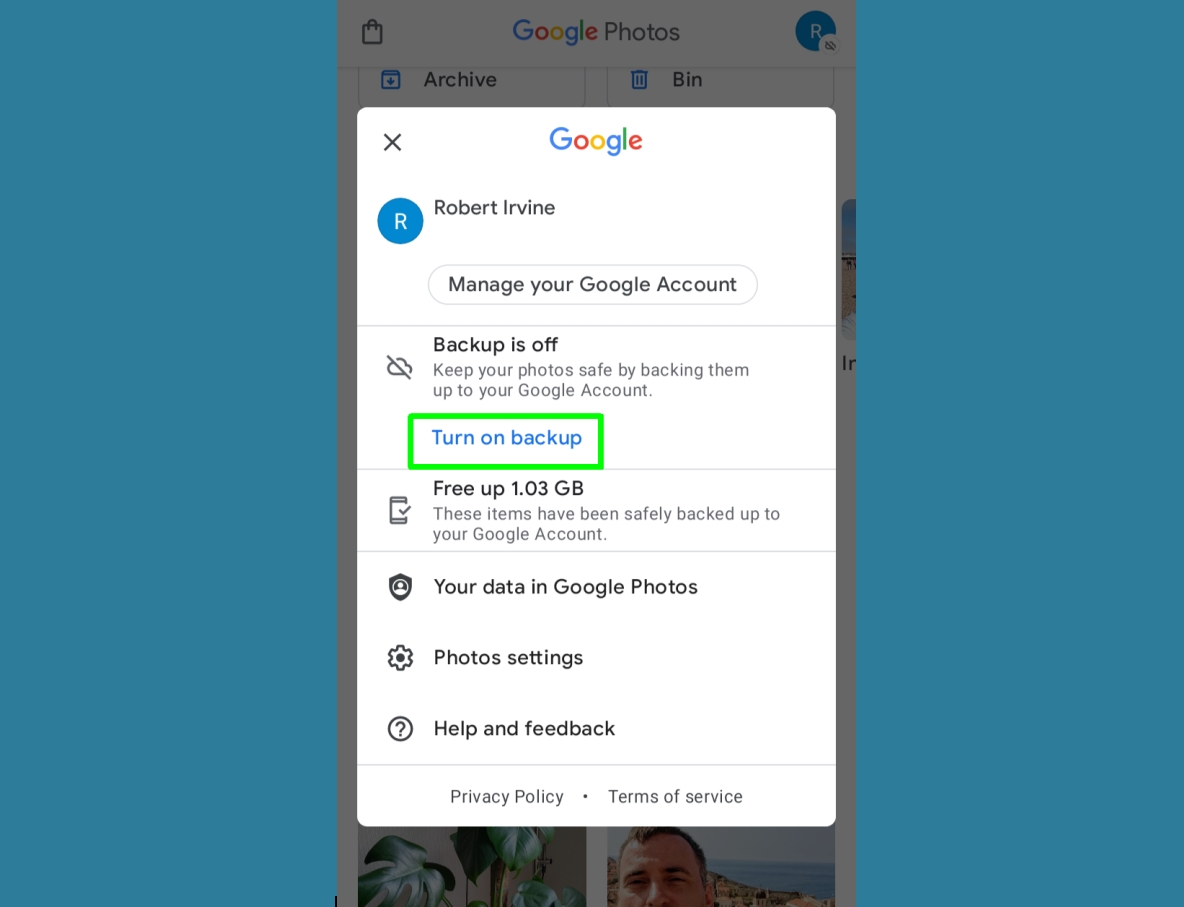The image features a gray smartphone with a blue background. On the screen, there is an interface displaying Google Photos. At the top of the screen is a shopping bag icon, followed by the colorful Google Photos logo with the characteristic colors of blue, red, yellow, and green. Below that is a blue circle containing a white "R," representing the user's profile, and icons labeled 'Archive' and 'Bin.'

In the foreground, there is a white popup box with a black "X" in the upper left corner, allowing the user to close the box. The box prominently displays the Google logo, followed by the blue circle with the white "R" and the name "Robert Irvine." Beneath this, there is a section prompting the user to "Manage your Google Account."

Further down, another box indicates that backup for Google Photos is turned off, along with a prompt: "Keep your photos safe by backing them up to your Google account." A green button with the text "Turn on backup" in blue appears below this message. Additionally, there is a small box offering to "Free up 1.03 GB" of space, assuring the user that these items have been safely backed up to their Google account.

At the bottom of the white box, there is another section labeled "Your data in Google Photos," which includes options for "Photo settings," "Help and feedback," a divider line, and links to the "Privacy Policy" and "Terms of Service." The background of the image shows portions of a couple of photos peeking out from behind the popup box.